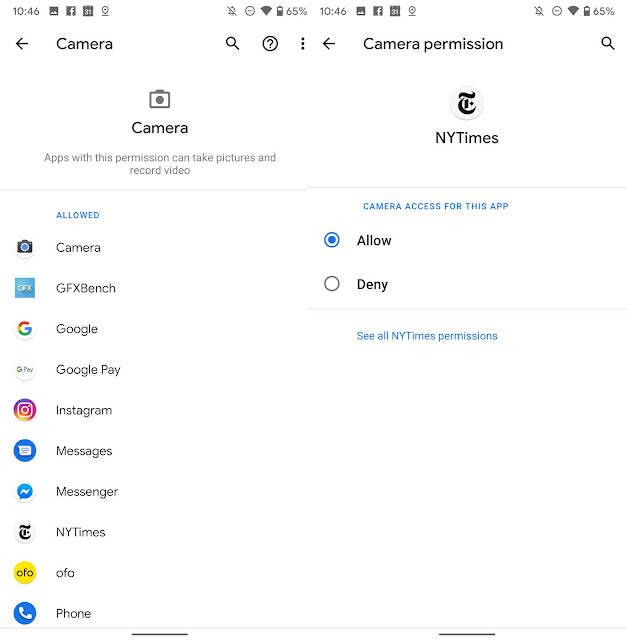Here's a cleaned-up and detailed caption for the described image:

---

**Detailed Description of a Device Permissions Screen:**

The image displays an enlarged view of a mobile device screen, potentially from a phone or tablet, showing the camera permissions settings.

At the top, the status bar includes several standard phone icons such as signal strength, battery percentage, and notifications. Below the status bar, there’s a navigation bar containing various icons: 
- A back arrow
- A camera icon
- A search (magnifying glass) icon
- A help (question mark in a circle) icon
- A vertical ellipsis (three dots) for more options.

The main section of the screen is divided into two parts:

On the left side, the screen lists apps with permission to access the camera. This section displays a camera icon followed by the text: "Apps with this permission can take pictures and record video." Below this, individual app icons are displayed alongside their names, including:
- The New York Times app (logo and name displayed as "NY Times")
- Camera
- GFX Bench
- Google
- Google Play
- Instagram Messages
- Messenger
- NY Times
- OFO
- Phone

Each app listed on the left side has a status shown in blue text, where "Allowed" is indicated next to permitted apps.

On the right side, specific permissions related to the New York Times app are detailed. The header states "Camera access for this app" in blue text. There is a toggle option below that allows the user to select "Allow" or "Deny" the permission, with "Allow" currently selected. Beneath this toggle, there’s an option labeled "See all New York Times permissions."

The design and icons are clearly aimed at managing and customizing app permissions for privacy and security purposes.

---

This caption provides a thorough and organized description, making it clear what is displayed on the screen.